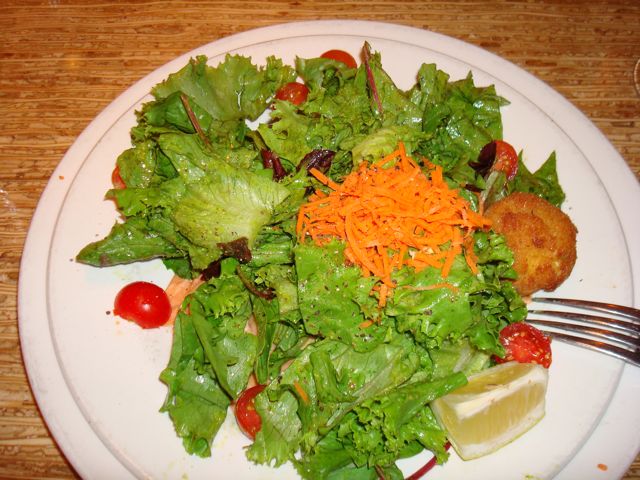This image features a close-up of a partially eaten, mixed salad presented on a plain, white round plate with a slightly curved-in bottom, set on a light wooden table. The vibrant salad showcases leafy green lettuce, bright orange slices of diced carrots, and halved cherry tomatoes in vivid red. A yellow lemon slice adds a citrusy touch, while elements of purple, possibly from purple lettuce or another ingredient, add more color. There is a solitary breaded or fried item that could be a piece of chicken or a crouton, adding texture to the dish. The salad is lightly dressed, and a fork lies face down to the right side of the plate. Despite the plainness of the plate, the fresh ingredients and variety of colors make the salad appear appetizing and simple yet appealing.